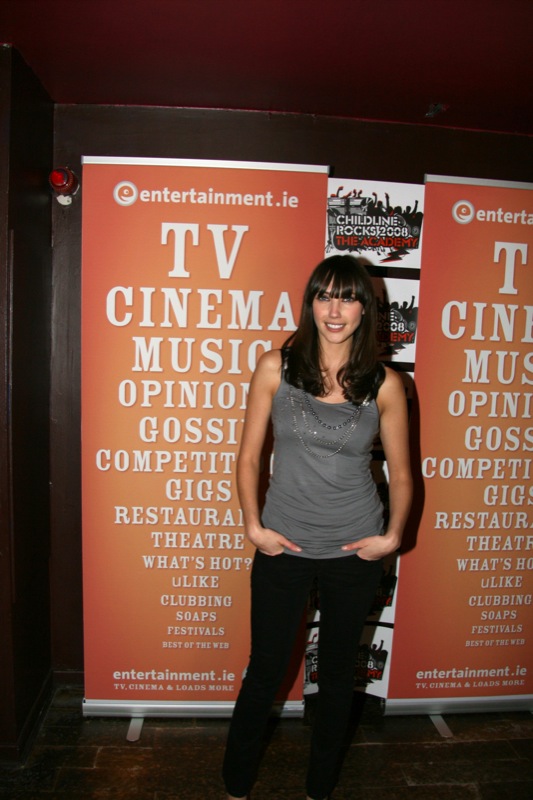This image features a light-skinned young woman, likely in her mid to late 20s, posing with a smile and looking directly at the viewer. She has dark brown hair that cascades over her shoulders. She is dressed in a sleeveless gray top that reaches her waist, paired with black pants, and accessorizes with two silver necklaces and a beaded lavender necklace. In the background, on either side of her, are two billboards with a reddish-orange hue. Both billboards display the text "entertainment.ie" at the top, followed by white letters listing "TV, Cinema, Music, Opinion, Gossip, Competition, Gigs, Restaurant, Theater, What's Hot, You Like, Clubbing, Soaps, Festivals," and additional smaller writing. Between these billboards, a third poster is partially visible, showing a white background with silhouettes and the text "Childline Rocks 2008."